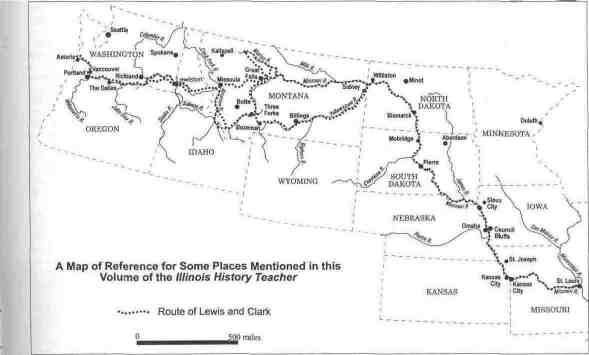The image is a black and white map from a textbook, depicting a partial map of the United States, specifically the upper northernmost and central regions, including the Midwest and parts of the West. The states visible are Washington, Oregon, Idaho, Montana, Wyoming, North Dakota, South Dakota, Minnesota, Iowa, Kansas, and Missouri. Each state is defined with dotted lines representing borders, while rivers are marked by wavy black lines. The map includes several major cities, including state capitals. There is a reference note at the bottom left corner: "A map of reference for some places mentioned in this volume of the Illinois History Teacher." A notable feature is the dotted line indicating the route of Lewis and Clark. Additionally, a solid black line at the bottom marks a scale from 0 to 500 miles, useful for measuring distances on the map. The overall appearance of the map, with its descriptive annotations and illustrative lines, suggests it is intended as an educational piece from a history textbook.